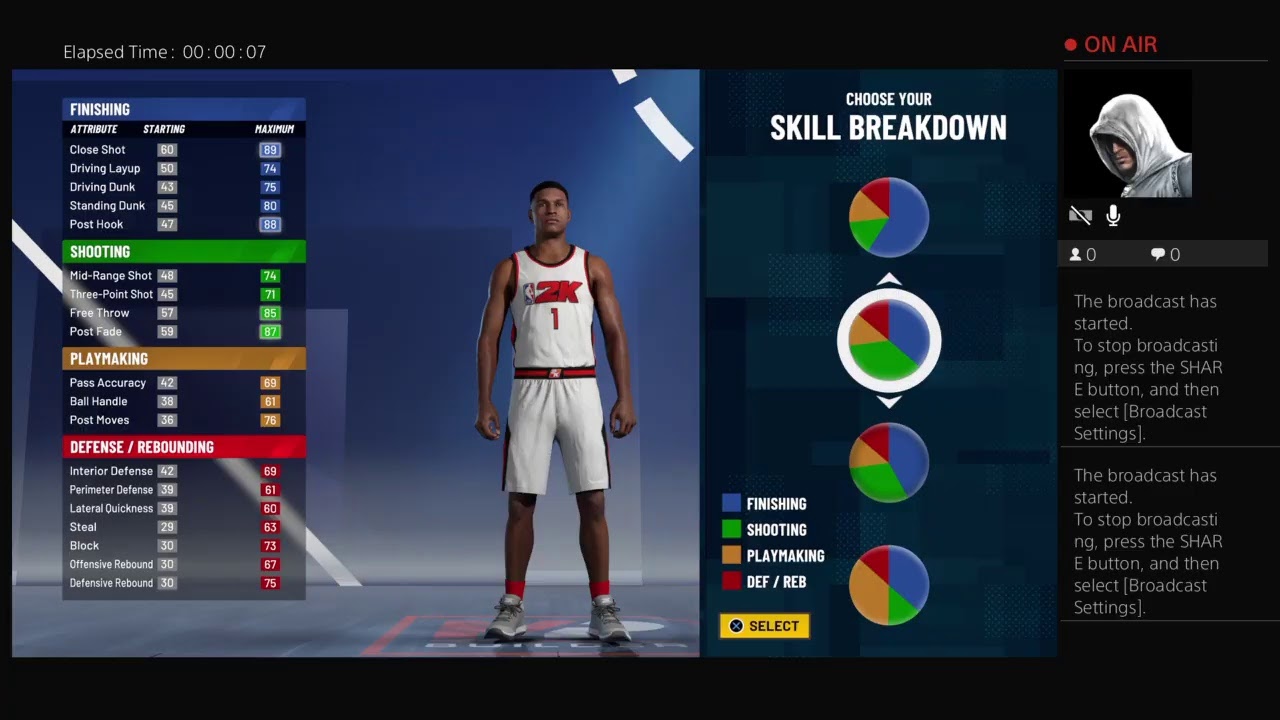The image features a detailed interface layout for a sports selection application. At the top, there is an elapsed time display reading "00:00:37". To the right, a "ON AIR" indicator is displayed in red, along with a red circle icon. On the left side of the image, a graphic of a basketball player demonstrates a finishing move, placed over a blue rectangle labeled "Finishing". Below it, there are three additional rectangles with accompanying information: a green rectangle labeled "Shooting", an orange rectangle labeled "Playmaking", and a red rectangle labeled "Defense/Rebounding".

At the center of the image, the text "Choose Your Skill Breakdown" is prominently displayed. Four pie charts are shown, each containing varying proportions of the colors blue, green, orange, and red, representing different skill sets. The second pie chart is selected, highlighted by a white circle around it. Below the pie charts, a table clarifies the color coding: blue stands for Finishing, green for Shooting, orange for Playmaking, and red for Defense/Rebounding.

Towards the bottom of the interface, there is a prominent yellow rectangle with the word "Select" on it. On the right side of the image, a person is visible, likely indicating a player ready to be chosen or edited within the application.